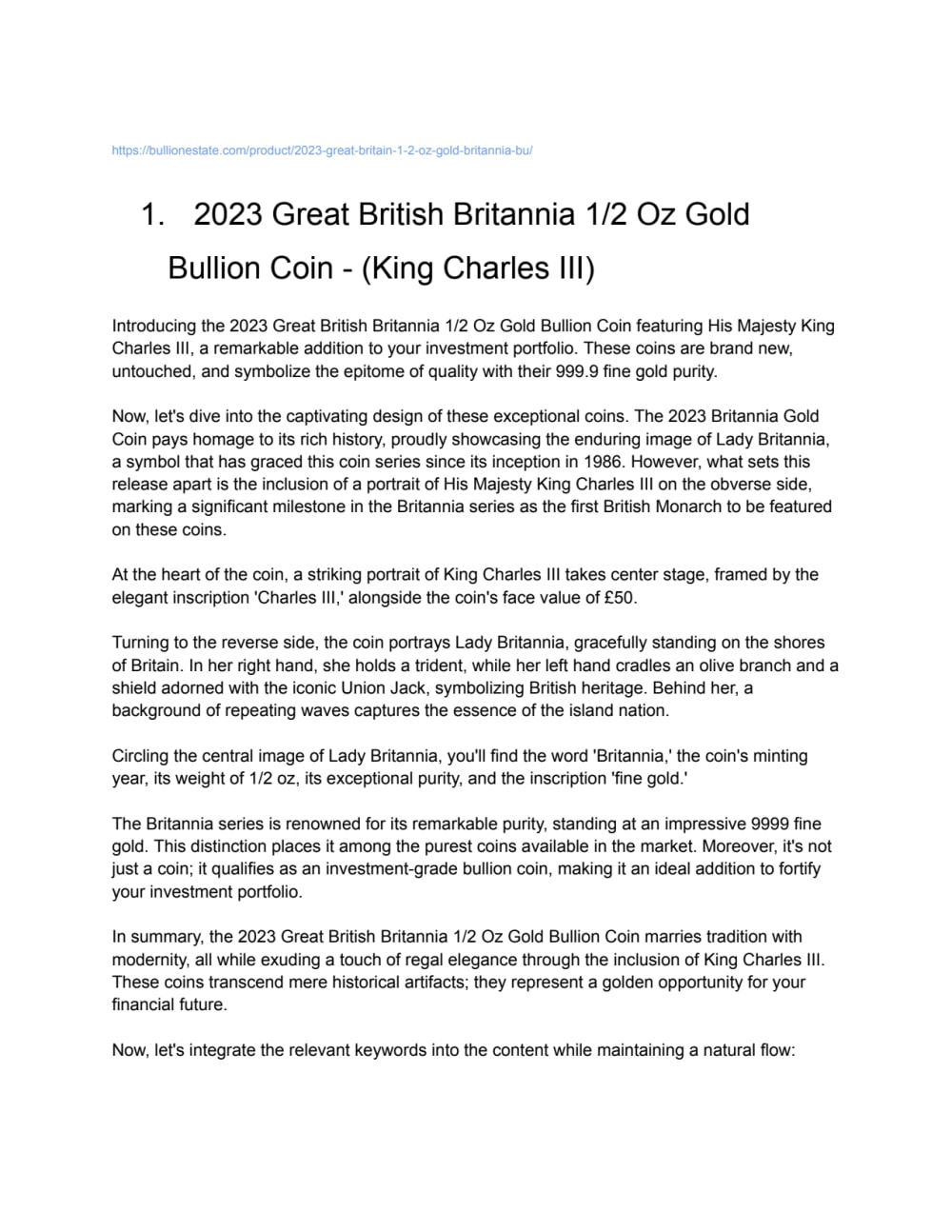The image is a detailed write-up discussing the 2023 Great British Britannia half-ounce gold bullion coin. It introduces this new investment opportunity, which features King Charles III on the obverse, marking a significant milestone as he is the first British monarch to appear on these coins. The text emphasizes the coin's premium quality, boasting 999.9 fine gold purity, and highlights its untouched, brand new status. It also delves into the design, paying homage to the enduring image of Lady Britannia on the reverse side, a symbol of British heritage that has adorned the Britannia series since 1986. The write-up underscores the historical and investment value of the coin, detailing its appearance and celebrating its $50 value. The promotional text aims to convince readers of the coin's merit as an investment, featured on bullionstate.com.